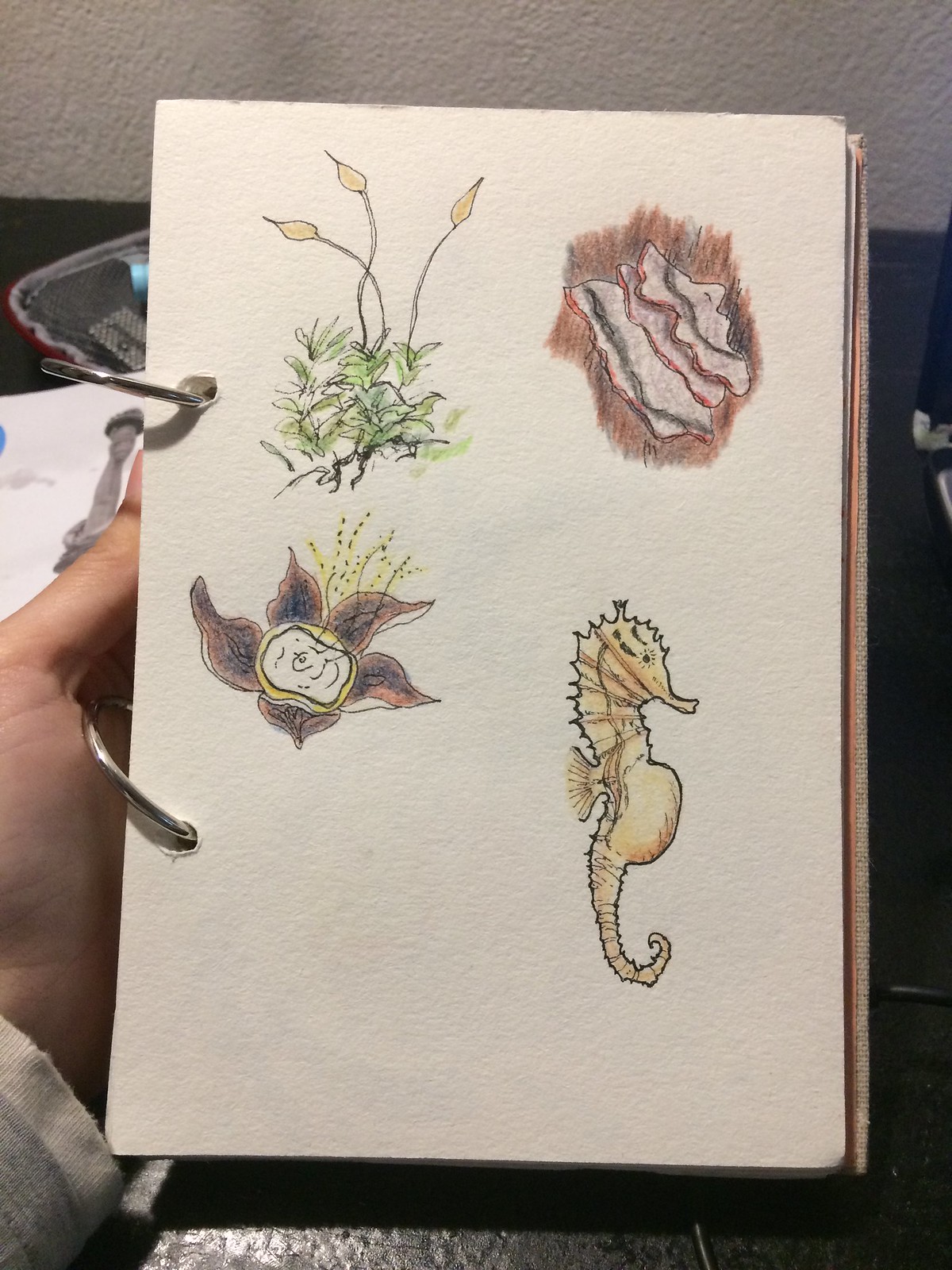In this detailed image of an artist's sketchbook, being delicately held by a human hand, we see four intricately colored sketches on the page. Positioned at the bottom right is a striking yellow seahorse, characterized by an extended belly, indicative of a male seahorse carrying eggs. Adjacent to the seahorse is a depiction that resembles an oyster or clam with its shell partially open, revealing the inner meat. The top left features a vibrant sketch of a flower with purple petals and yellow insides, capturing the delicate beauty of a blossoming bloom. Nearby, a green plant emerges, adorned with yellow flowers, possibly water lilies or irises, with three bulbs and a backdrop of lush green foliage. Dominating the upper right corner, there's a brown, layered stone, adding a rugged, natural element to the collection. The sketchbook, bound with two large wire rings, rests on a desk with a black top, with some indistinct items visible beyond the journal.